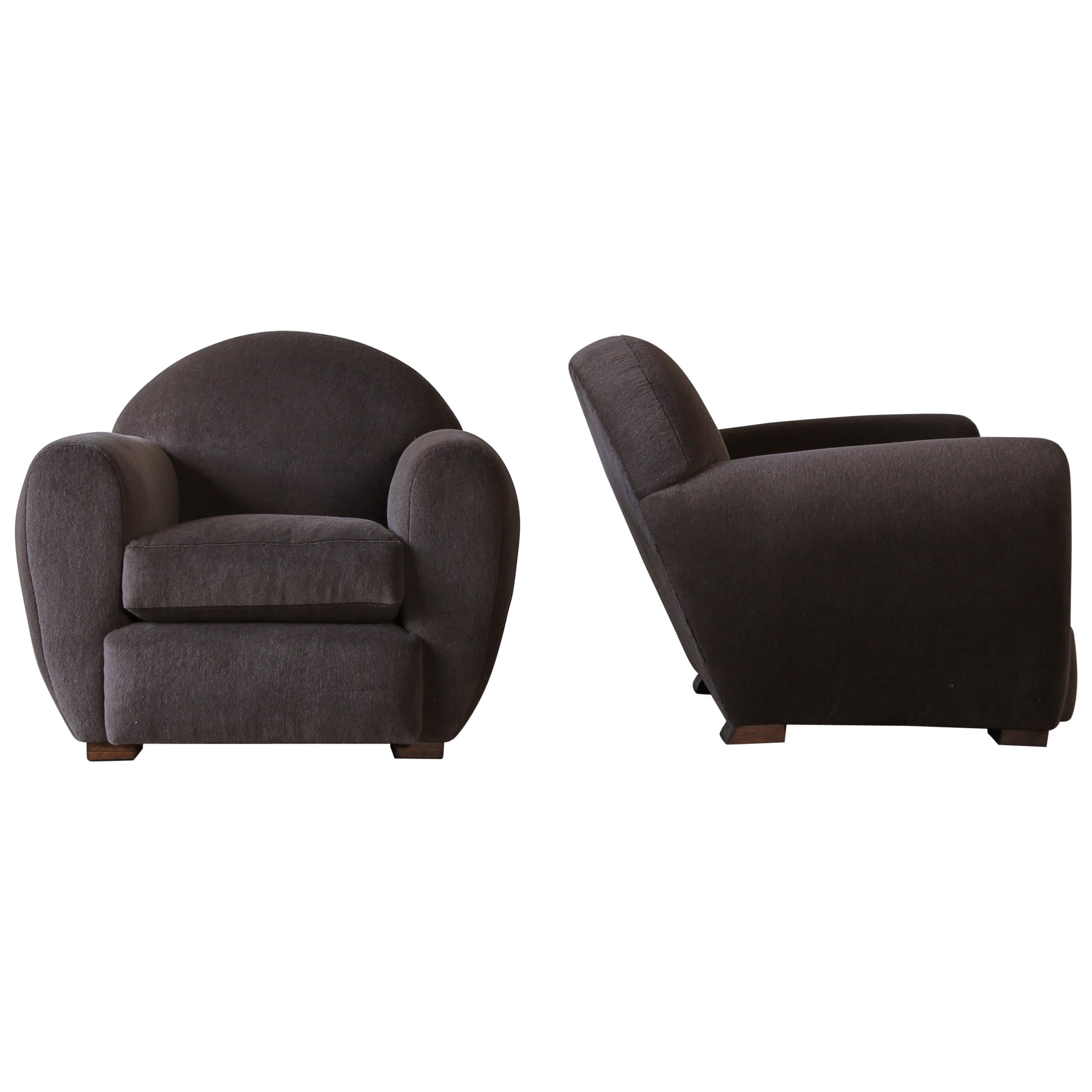This image showcases a gray armchair designed for a living room, displayed in two different orientations against a plain white background. The chair features a low, curved backrest and thick armrests, providing a sense of comfort and robustness. It is upholstered in a gray fabric, the specific type of which is not identified. 

The left side of the image displays the chair facing forward, revealing a plush seat cushion and a secondary structural layer beneath it for added support. The chair stands on elegant wooden legs, which complement its overall aesthetic.

The right side of the image presents a side view of the same chair, highlighting the substantial armrest and a portion of the curved backrest. This view also offers a glimpse of the wooden legs supporting the chair, further emphasizing the design continuity.

The setting is minimalist, with a plain white background and no text, keeping the focus solely on the armchair's design and structure.